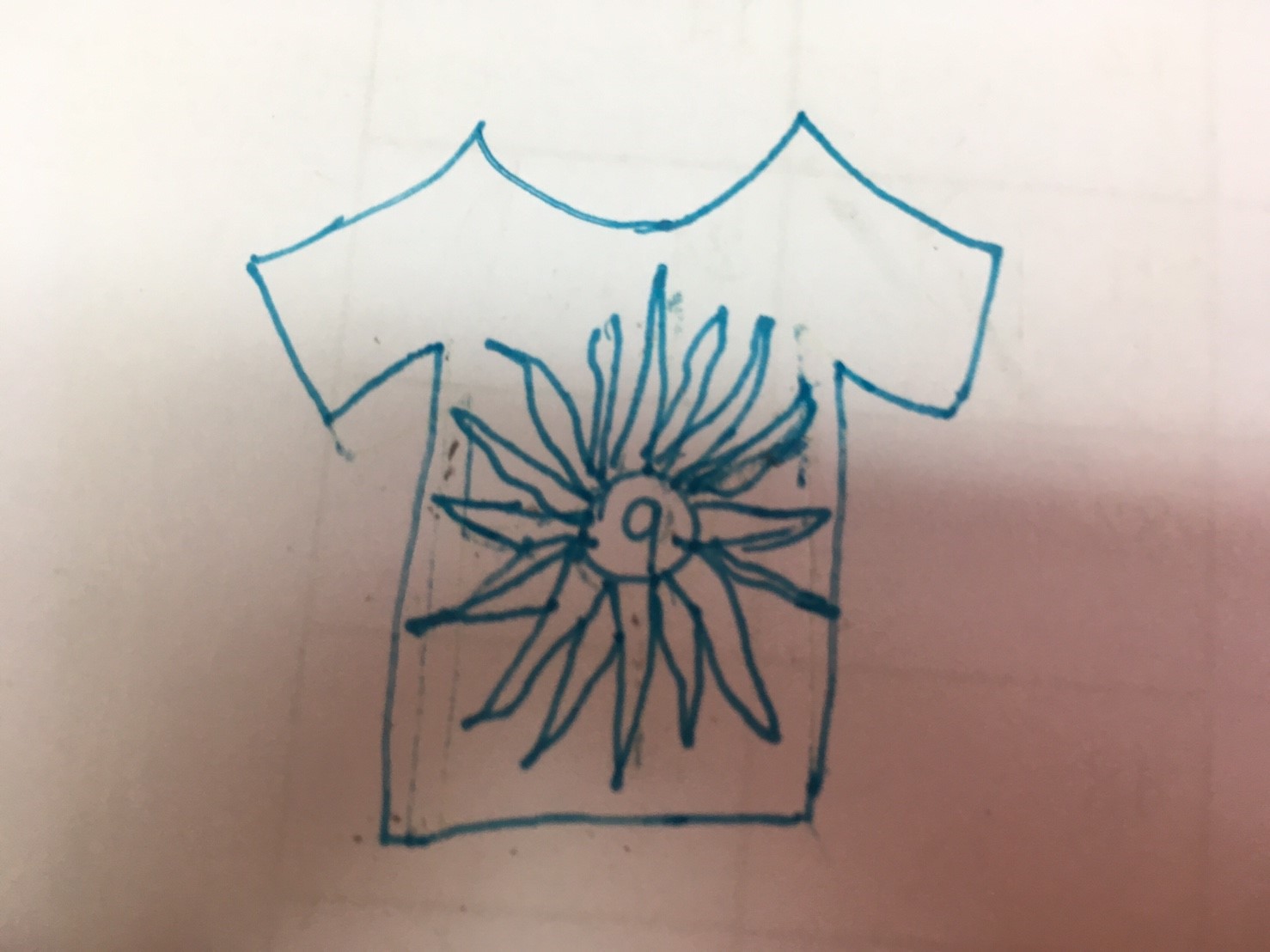The image is a detailed hand-drawn sketch of a short-sleeve, rounded collar graphic shirt, created using a blue marker. The design has not been filled in with color; only the outlines are depicted. Dominating the front of the shirt is an intricate sun or flower motif, characterized by numerous triangular shapes radiating from a central circle with an additional smaller circle at its heart. This drawing is placed on a white sheet of paper. Through the shadows on the bottom half of the page, the outlines of rectangles on an underlying sheet are faintly visible. The photograph also captures the hand of the artist and the device used to take the picture, contributing to the composition. The overall form of the image is rectangular, with its top and bottom sides longer than its left and right sides.